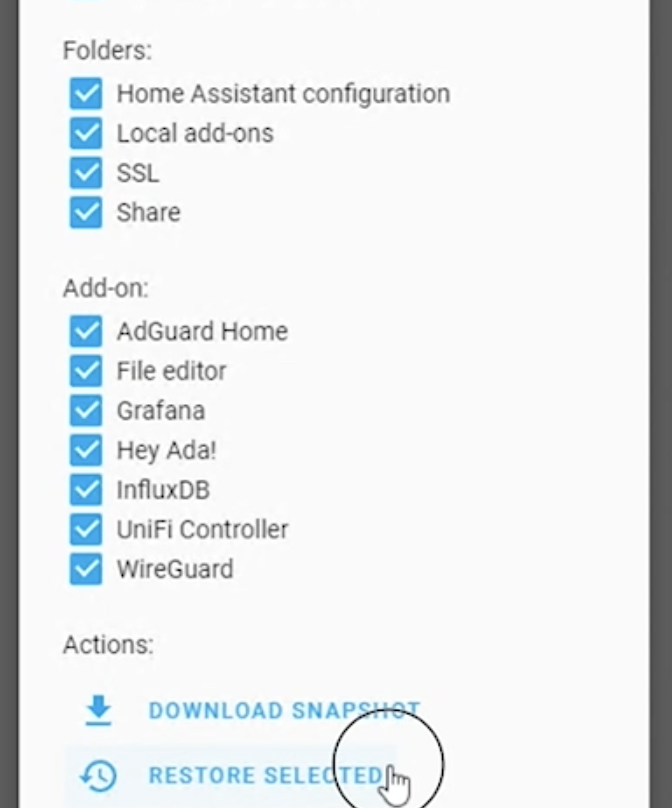The image is a screenshot captured from a device, possibly a tablet, smartphone, desktop, or laptop. The background is predominantly white, with dark grey or black bezels, while the top edge of the screen is entirely black. At the top, the black text "folders" is displayed. Following that, it features "dot dot," indicating some additional content.

Below this header, four dark blue squares with white check marks are present, labelled as follows: "Home Assistant Configuration," "Local Add-ons," "SSL," and "Share." A small space separates these from the next section.

Next, a title in black text reads "Add-ons." Each of the following entries next to this title has a blue box with a white check mark:
- AdGuard Home (with "A", "G", and "H" capitalized)
- File Editor ("F" capitalized)
- Grafana (spelled "G-R-A-F-A-N-A" with "G" capitalized)
- HeyAta ("H" and "A" capitalized; "Ata" is spelled "A-D-A" with an exclamation mark)
- InfluxDB ("DB" capitalized)
- UniFi Controller ("U" and "F" capitalized; spelled "U-N-I-F-I")
- WireGuard ("W" and "G" capitalized)

Under this list, the section "Actions" is displayed in black text, followed by a "dot dot." A downward-pointing arrow directs attention towards a flat blue line. This blue line is connected to a bold blue text reading "DOWNLOAD SNAPSHOT" in all capital letters.

Directly beneath this, an icon of a clock with an arrow circling almost entirely around it appears in blue. To the right of this icon, the text "RESTORE SELECTED" is displayed in all capitals, framed by a light blue box. Finally, on the far right side of the image is a black circle containing a white hand, completing the interface description shown in the screenshot.